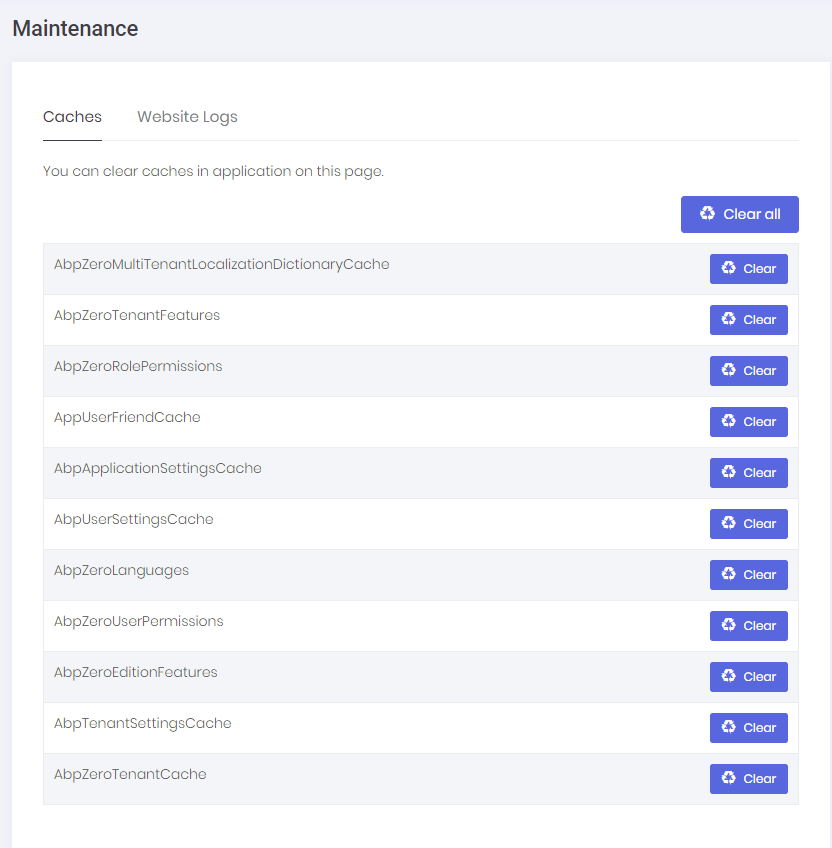The image displays a maintenance interface. At the top, there's a light gray header labeled "Maintenance." Below it, the background transitions to white. On the left side, the word "Caches" is prominently displayed with a line beneath it. To the right of this section, the phrase "Website Logs" appears, with a lighter-colored line extending horizontally under it, reaching the far-right side of the image.

Below these headers, the page informs users that they can "clear cache and application on this page." Subsequently, there is a series of rectangular sections that alternate between light gray and white backgrounds. Each section has a rectangular blue button labeled "Clear" positioned on the right side.

From top to bottom, the sections contain the following labels:
1. ABP Zero Multi-Tenant Localization Dictionary Cache
2. ABP Zero Tenant Features
3. ABP Zero Role Permissions
4. ABP User Friend Cache